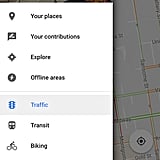A cropped and slightly blurry screenshot from an unspecified navigation software, potentially Google Maps, revealing an obscured map partially covered by a white background navigational menu located on the left-hand side of the screen. The menu features multiple options segmented into different categories. The first section includes: "Your Places," "Your Contributions," "Explore," and "Offline Areas," written in black text on a white background. The second section displays options for "Traffic," "Transit," and "Biking," with "Traffic" being highlighted with a grey background and blue text, while the others remain in black text. The text and background in the screenshot are blurred, making finer details difficult to decipher. The faintly visible map in the background offers no clear indications of its location due to the overlay and cropping.